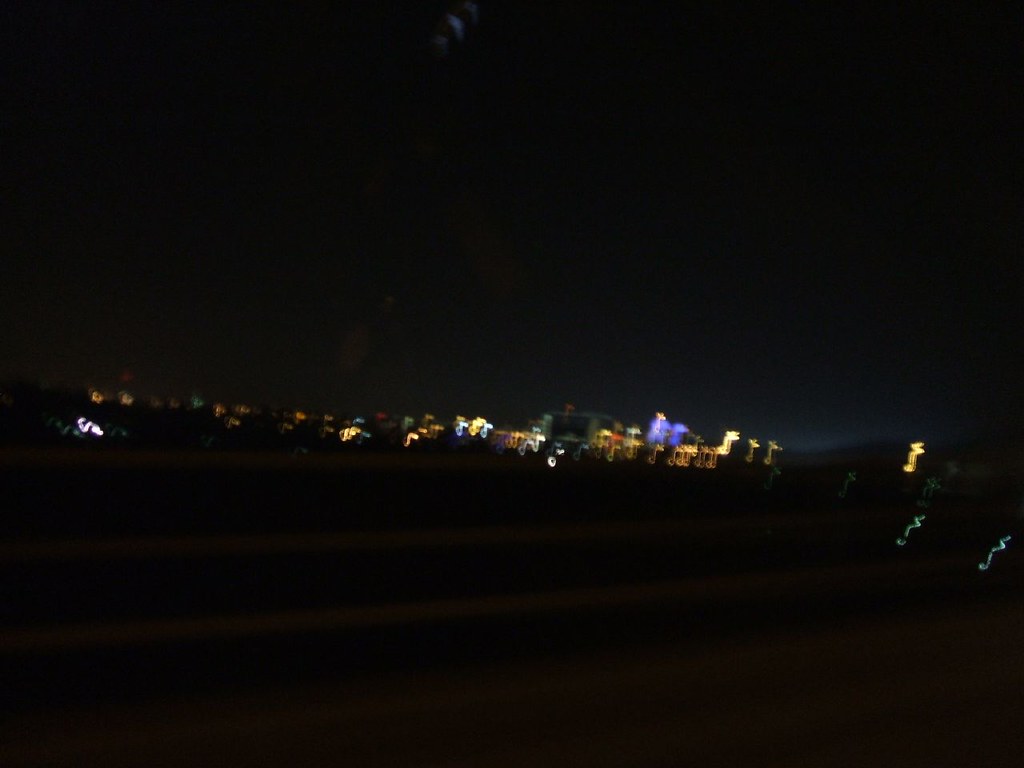Blurry nighttime photograph of a distant cityscape, capturing the essence of a bustling urban environment under a dark sky. The image, taken while either the photographer was in motion or due to a sudden drop of the camera, showcases a city bathed in a mix of bright lights and shadowy corners. Despite the blurriness, the illuminated buildings, shops, and houses are discernible, with streaks of car headlights contributing to the overall vibrancy. A faint glow, possibly light pollution, casts a subtle aura around the city. In the foreground, what appears to be rippled sand adds a textured contrast, potentially enhanced by the blurry effect of the lights. This photograph encapsulates the dynamic and transient nature of nighttime in an urban setting.